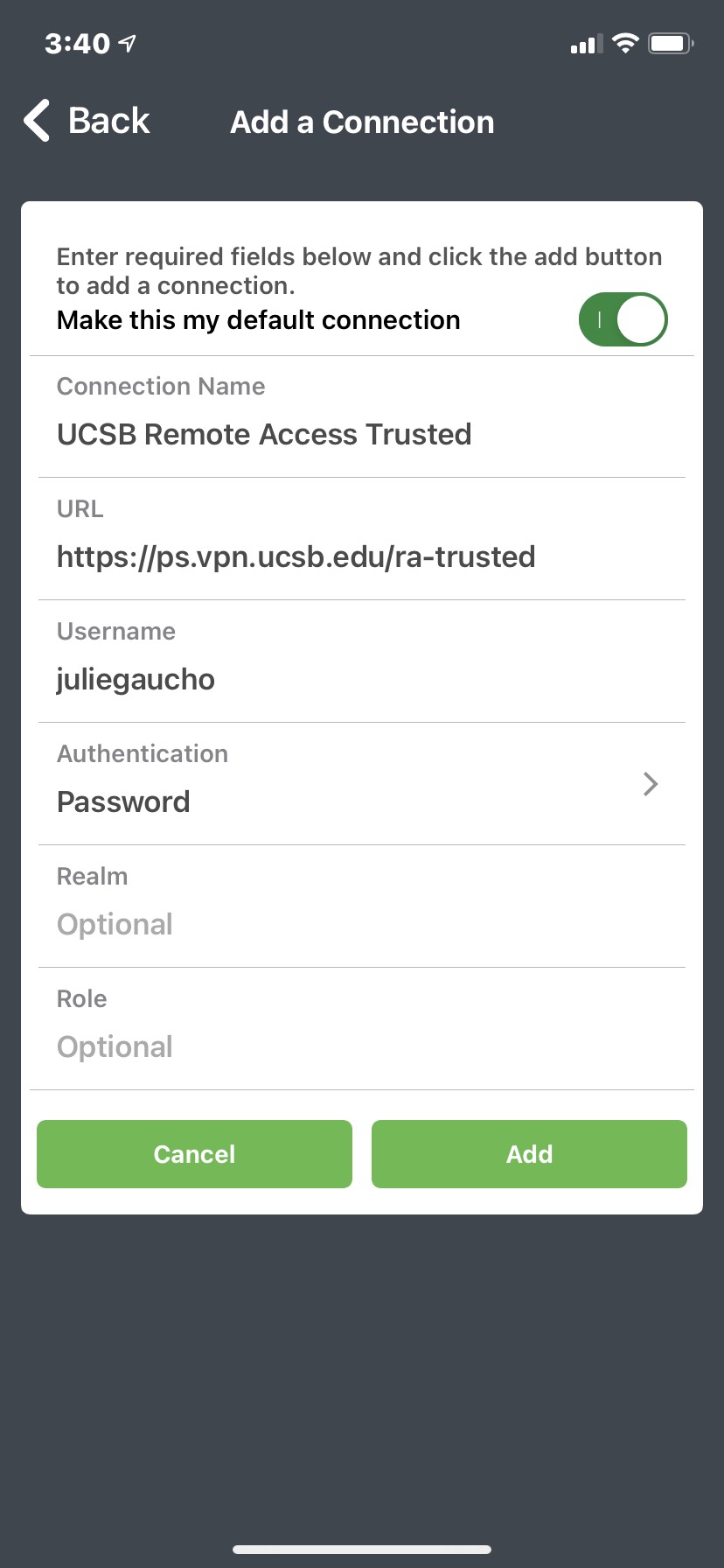This detailed image captures a smartphone screen displaying a configuration page for adding a new network connection. The background of the screen is black.

At the very top, the status bar includes:
- The time, which reads "3:40" in white numbers.
- An icon of a small arrow pointing to approximately 2 o'clock.
- On the far right, there are three out of four bars highlighted, indicating strong wireless signal strength.
- A horizontal battery icon nearly filled to denote an almost full battery.

Below the status bar, the next section showcases navigation and the current page title:
- A white left-pointing caret with the word "Back" next to it.
- Centered on this line is the title reading "Add a Connection".

The main content occupies a white rectangular area in portrait orientation. The information fields displayed are as follows:
- A prompt stating: "Enter required fields below and click the add button to add a connection."
- An option, "Make this my default connection," with a toggle switch shown as dark green with a white button positioned to the right, indicating it's turned on.
- The field labeled "Connection Name" filled with "UCSB Remote Access Trusted."
- A field labeled "URL," displaying: "https://ps.vpn.ucsb.edu/ra-trusted."
- A "Username" field filled with "Julie Gaucho."
- An "Authentication" field with the input labeled as "Password." A right-facing caret next to this word suggests additional configuration options.
- A field labeled "Realm," with "Optional" noted beneath it.
- A field labeled "Role," also with "Optional" beneath it.

At the bottom of the white rectangle, there are two green rectangular buttons:
- The left button labeled "Cancel" in white font.
- The right button labeled "Add" in white font.

Below this section, the remainder of the screen is black.